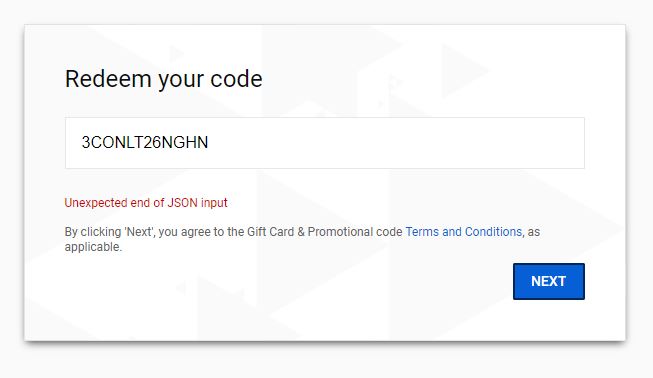In the image, there is a pop-up window with a white rectangular background, oriented horizontally. At the top, in the largest font and in black, the text reads "Redeem Your Code." Below this title, there is a data input field with a gray outline containing the code "3CONLT26NGHN" in black text.

Directly underneath the input field, a message states, "An unexpected end of JSON input. By clicking Next, you will read the Gift Card and Promotion Code terms and conditions as applicable." The phrase "terms and conditions" is highlighted in blue, indicating it is a clickable link.

At the bottom right corner of the pop-up, there is a blue "Next" button with a black outline, and the word "Next" is written in white. The overall color scheme of the pop-up includes black, white, blue, and various shades of gray, with the background being a very light gray.

This pop-up appears to be a feature intended for entering and redeeming a promotional or gift card code, though its specific platform (desktop, mobile, or tablet) is not indicated.